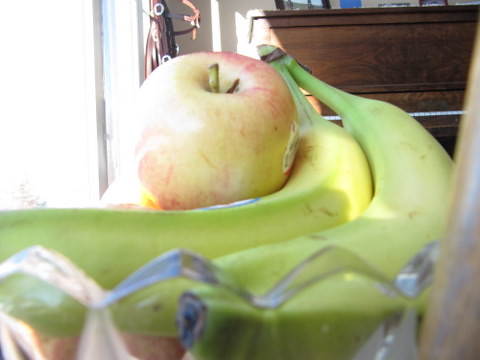In this close-up photograph, the central focus is a glass bowl filled with fruit, prominently placed in a setting that exudes a cozy, domestic ambiance. The bowl, intricately designed with triangular points that soften into rounded edges, holds two bananas with greenish peels, suggesting they are underripe. Nestled beside them is a yellow apple tinged with hints of red, featuring a small white sticker and a green stem.

The background reveals a diverse array of household elements, detailed in a thoughtfully composed arrangement. A sliding glass door allows an almost blinding bright light to flood the scene, casting a warm glow that bathes the room in sunlight. Adjacent to the door, a coat rack supports a brown bag, subtly blending into the background.

To the right, a brown wooden piano comes into view, showcasing a polished wood grain with shades of light and dark brown. The white piano keys contrast against its body, with just a hint of a tan-colored wall behind the instrument, adding depth to the photograph.

The entire setting creates a harmonious balance between the fruits in the foreground and the homey elements in the background, capturing a moment of everyday beauty.